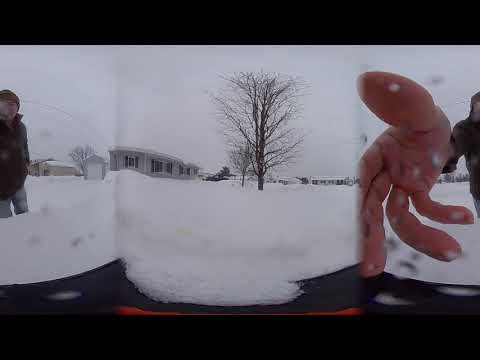In a panoramic outdoor scene stretching 360 degrees across the frame, the image captures a stark and cold winter day with deep, white snow covering the ground up to knee-level. The skies are a somber gray, emphasizing the chill in the air. Central to the image stands a barren tree, devoid of leaves, its branches reaching upwards in stark contrast to the overcast sky.

On both the left and right edges of the panorama is the same man, appearing twice due to the panoramic effect. On the left, he stands almost undistorted, dressed in heavy, dark winter clothing and a hat, partially obscured by the snow banks. To the right, he reappears, his arm outstretched towards the camera with a dramatically enlarged hand dominating that side of the image due to the perspective distortion.

In the background, a couple of naked trees dot the snowy landscape, and one-story houses are visible under the horizon, hinting at a residential area. A shiny black metallic object, unidentifiable, stands in the near foreground, adding a touch of mystery to this serene yet stark winter scene.